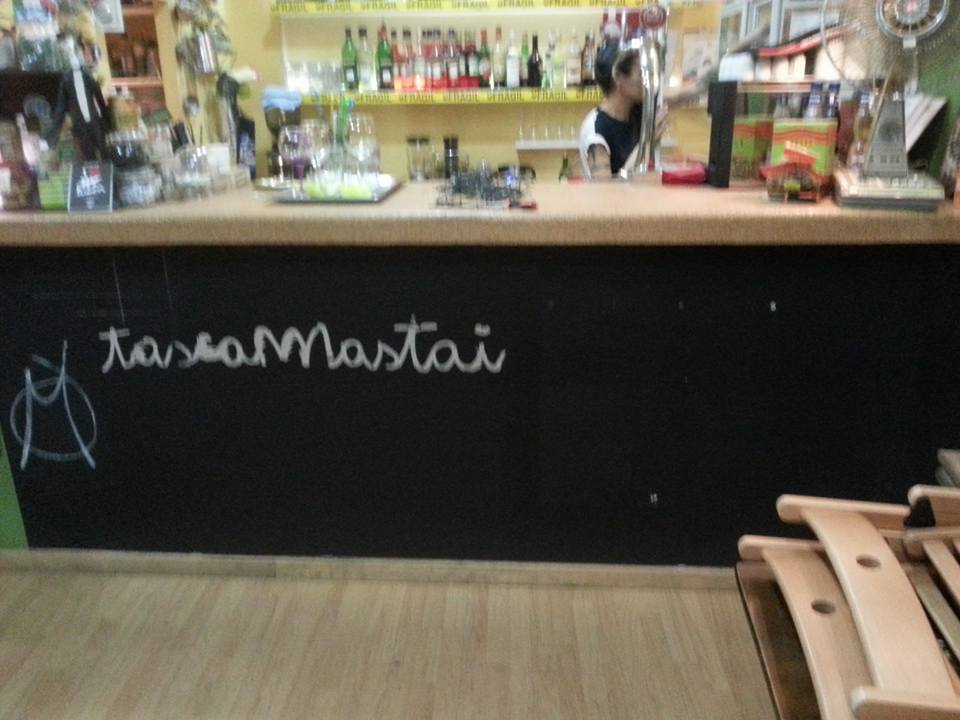In this image, set in a restaurant bar, a variety of objects are captured in detail. Dominating the scene is the central black wall of the bar counter, emblazoned with the word "TASCOMLASTAI" in white letters. A woman stands behind this counter, clad in a black and white short-sleeved T-shirt, positioned just behind a silver metal bar. Behind her is a shelf filled with numerous wine bottles, adding a vibrant mix of colors, primarily reds and greens, to the background. On the bar counter itself, there are several wine glasses arranged in the center, while on the right side of the counter, a fan rests. The floor extends from the bottom, transitioning into the wooden structures and the full counter setup in the middle of the composition. The overall photo, although somewhat blurry, presents a vividly busy and richly colored bar scene, with details that point to a lively and well-stocked environment.